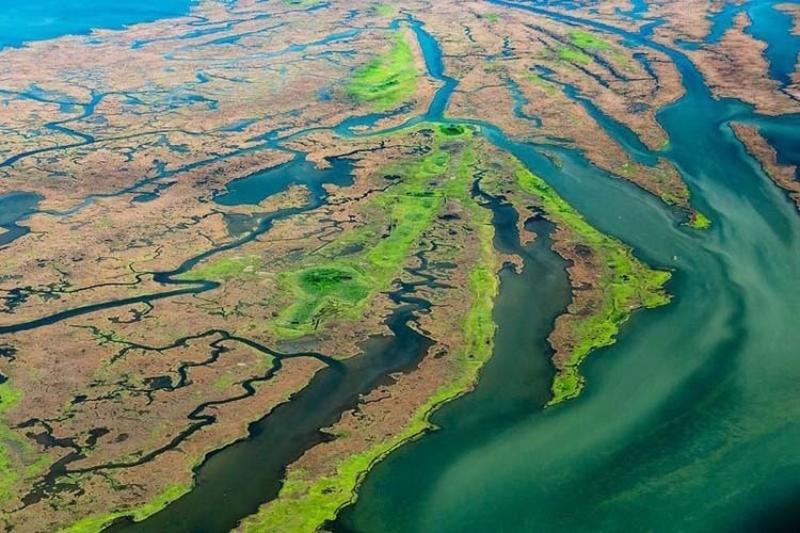This aerial photograph showcases a striking view of a vast lagoon or marshy coastal region, possibly near the mouth of a significant river like the Mississippi. The landscape is an intricate tapestry of brown and green vegetation interspersed with winding waterways. The land appears patchy and marsh-like, often dark brown with blotches of green algae. The water, in shades of dark emerald green and lighter blue, weaves through the land in squiggly lines and diverse shapes, creating a natural artwork. From an elevated perspective, perhaps from an airplane, the image captures the raw beauty of this uninhabited area, where nature's palette paints a seemingly abstract masterpiece of land, water, and algae.